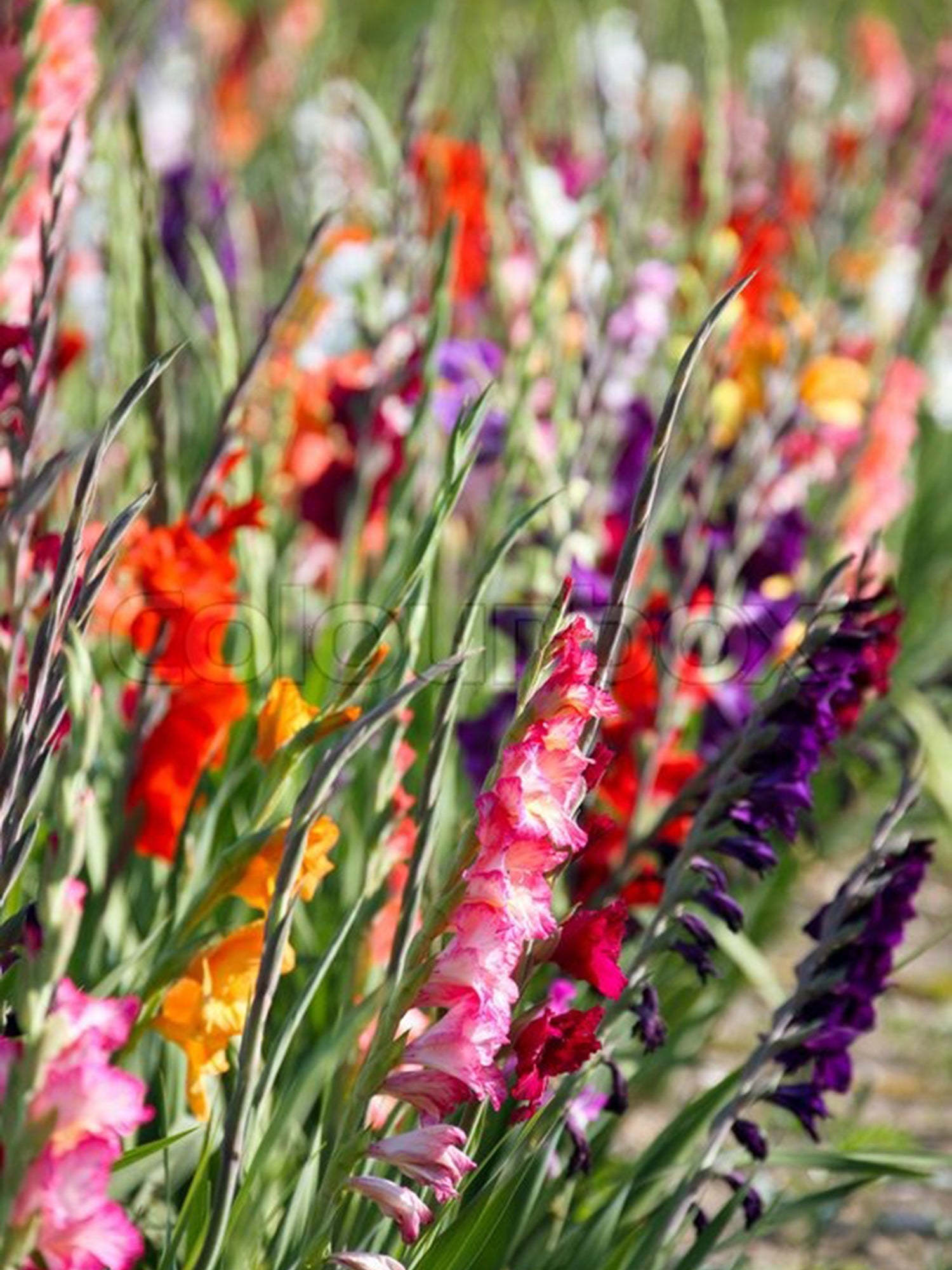The photograph captures a vibrant field of gladiolas during the daytime. Viewed from a low angle, it showcases a striking array of flowers, each attached to slender, spiraling stems. These flowers exhibit a stunning variety of colors including bright magenta, purple, pink with white centers, orange, and gold. Most prominently, magenta and purple flowers are located towards the center-bottom of the image, whereas the top features more fully bloomed flowers, transitioning to buds at the bottom. As the eye moves towards the background, the flowers gradually blur, creating a depth effect. Subtle yet distinct, the watermark "COLOURNOOX" is embossed across the center, hinting at the likely copyright owner of the image.